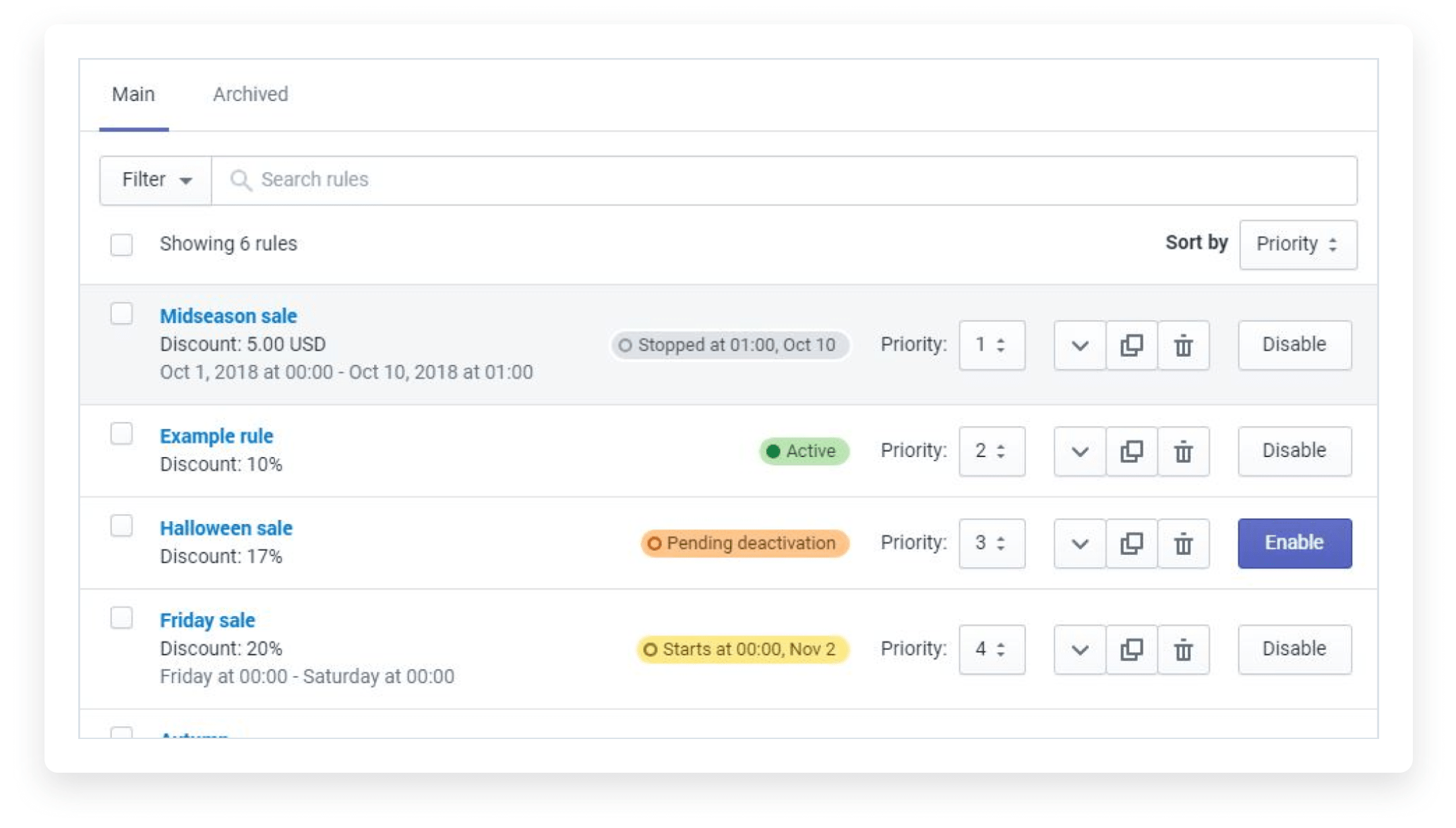**Screenshot of Rules Management Web Page**

The screenshot displays a well-structured, landscape-oriented web page. At the top, two tabs labeled "Main" and "Archived" are positioned side by side. The "Main" tab is highlighted with black text and a blue rectangle beneath it, indicating it is the active selection.

Below the tabs, a navigational bar contains a search box with the placeholder text "Search Rules" accompanied by a magnifying glass icon. Adjacent to this is a drop-down box labeled "Filter." 

Directly beneath this bar, a rectangular notification states "Showing six rules." To the left of the rules list, there are blank checkboxes presented in linear rows for selection.

On the right-hand side at the top, a sorting feature is visible with an option set to "Sort by: Priority" from the drop-down menu.

The rules are listed as follows:

1. **Mid-Season Sale** (in blue font) 
2. **Example Rule** (in blue font)
3. **Halloween Sale** (in blue font)
4. **Friday Sale** (in blue font)

Each title is followed by detailed rule descriptions in black font. Beside these titles, colored tags indicate different priority levels: gray, green, orange, and yellow, each with rounded edges. Additionally, there are functional buttons provided to enable or disable the respective rules.

This comprehensive layout facilitates easy navigation and management of rules.